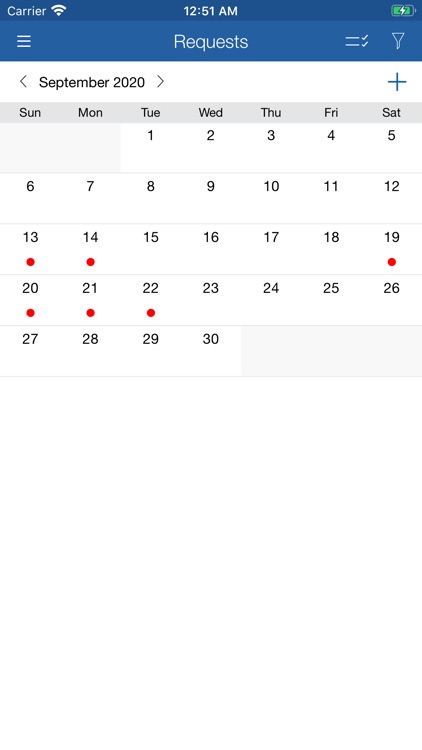This image, set against a white background, depicts a screenshot of a smartphone calendar application interface. At the top of the screen is a blue status bar. In the upper left corner of this bar, white text displays the word "carrier." To the right of this text is the Wi-Fi signal icon, and centrally positioned at the top is the time, shown as 12:51 a.m. In the upper right corner, a battery icon indicates a full charge.

Below the status bar, in the center of the screen and in white text on a blue background, the word "Requests" is displayed. Adjacent to "Requests" are two short horizontal lines with white check marks to the right.

Directly beneath this, against the main white background, is a bold black text header reading "September 2020," accompanied by a plus sign (+) on the far right. Underneath this header is a gray banner that lists the days of the week from left to right: Sunday, Monday, Tuesday, Wednesday, Thursday, Friday, and Saturday.

Occupying the space below the gray banner are the dates of the month, laid out in a grid format from the 1st to the 30th. Notably, the dates 13th, 14th, 20th, 21st, and 22nd are marked with red circles, indicating special notes or events on those days.